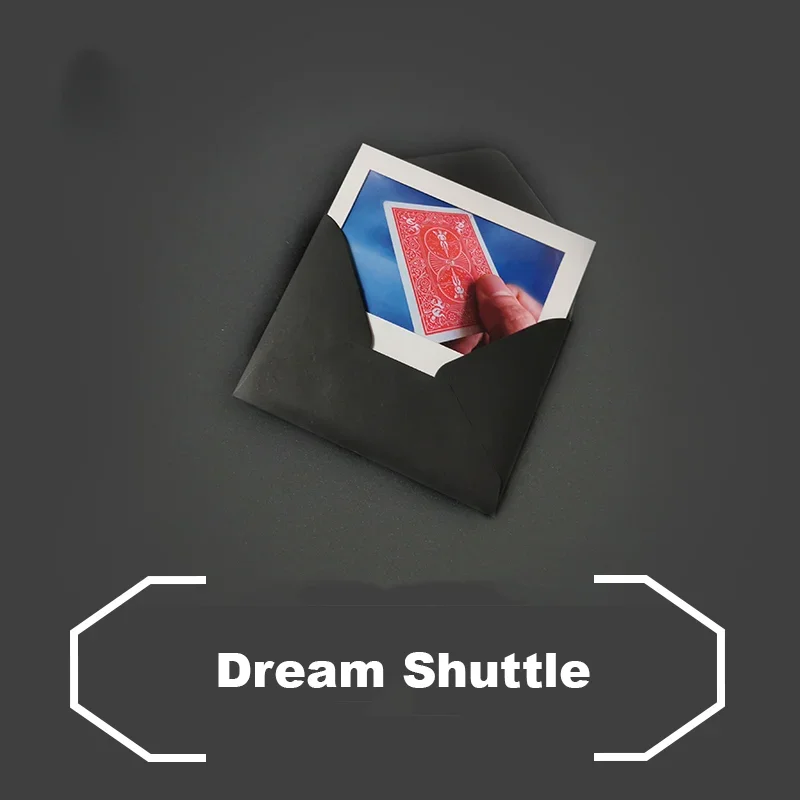The image features an advertisement set against a charcoal black background, showcasing a partially opened black envelope. Inside the envelope is a white card, revealed about halfway, with a vibrant blue painted rectangle on its cover. The focal point of the card is a vivid red playing card, bordered in white, depicting two angels. This playing card is held delicately by a person's right hand, with only the thumb and index finger visible, gripping the card's right corner. Below this striking visual, the phrase "DREAM SHUTTLE" is prominently displayed in capital letters, encased within white brackets resembling half of a pentagon. The ad's sophisticated color palette includes shades of black, white, red, and blue, creating a visually compelling and eye-catching design.